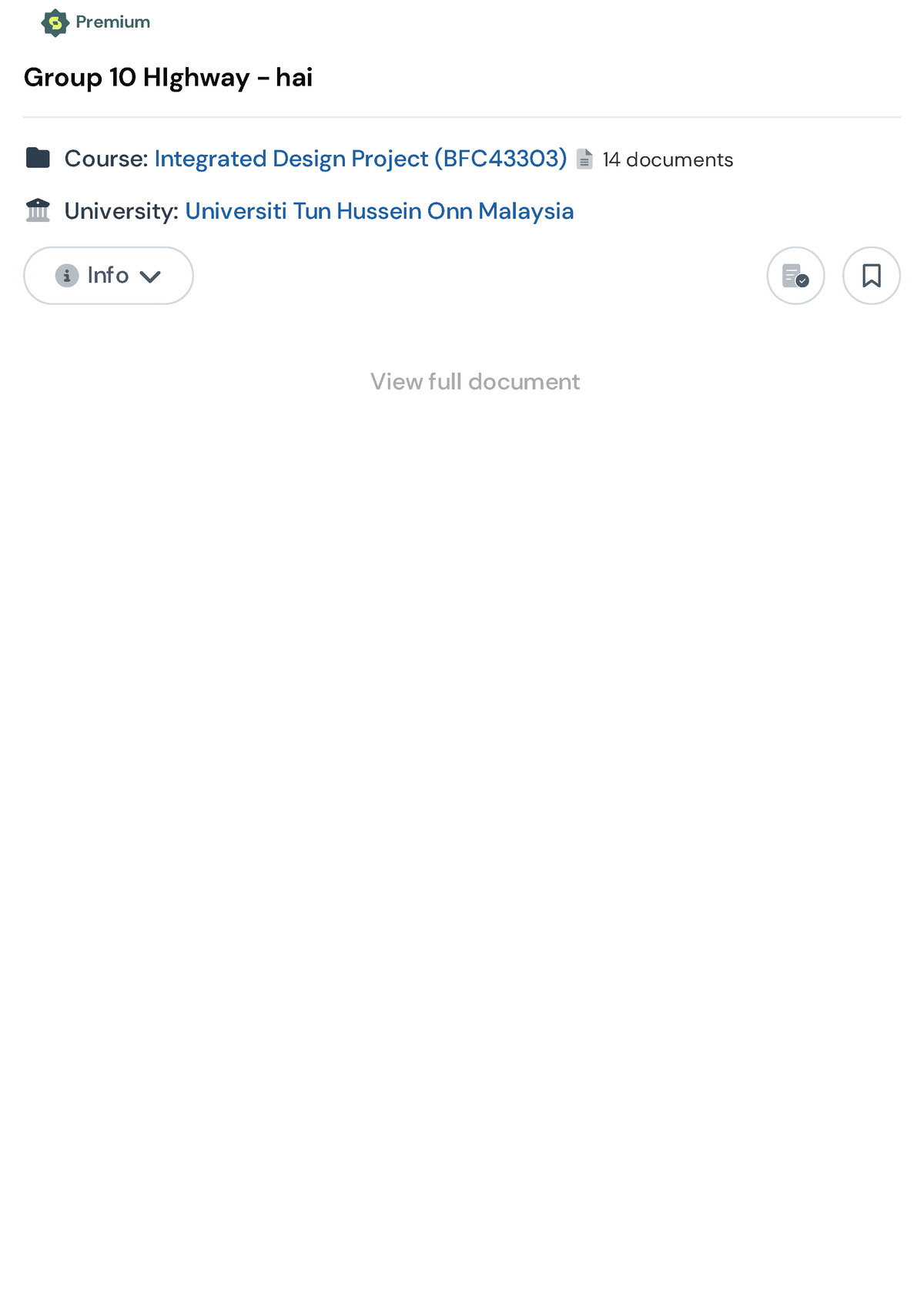This digital screenshot prominently features a user interface from an educational platform. In the top left corner, a gray and green star-shaped logo is displayed, with the word "Premium" adjacent to it. Directly beneath, the text reads "Group 10 Highway - HAI," indicating a specific group or category. Following this, there's a section titled "Course" accompanied by a small blue file folder icon labeled "Integrated Design Project," with the course code "BFC 43303" next to it. Below this title, it notes "14 documents," suggesting the number of files available in this course. Toward the bottom, a logo of a university is seen, labeled "Universiti Tun Hussein Onn Malaysia." Finally, a dropdown button with a downward arrow and the word "Info" is located near the university logo.